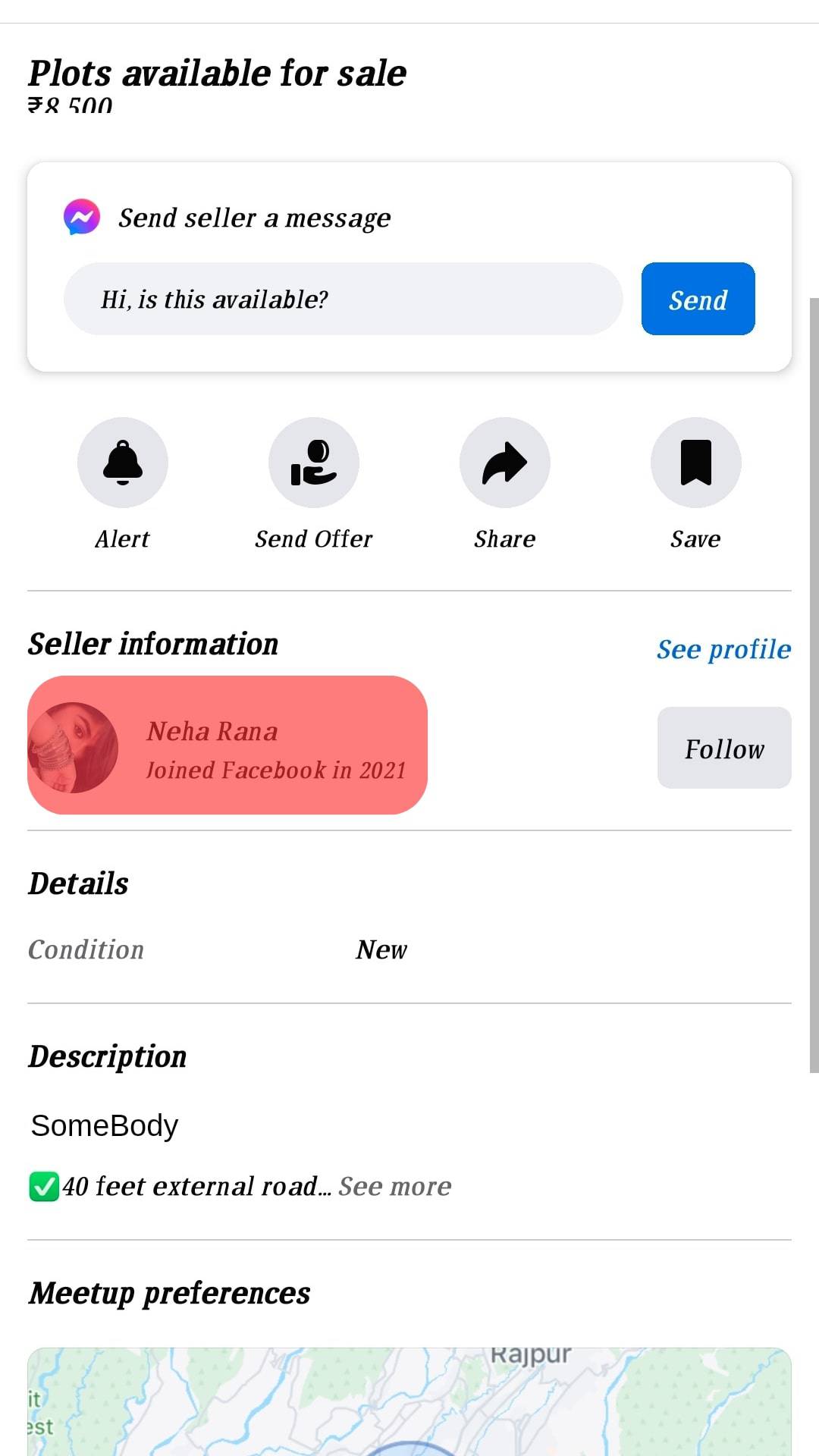In the image, the top left corner prominently features the text "Plots available for sale" in black-colored font. Directly underneath this text, the price "8500" is displayed, though the currency is not specified. Below the price, there is a rectangular button labeled "Send Seller a Message" with a small messenger-like icon to its left. This icon features a gradient of purplish, bluish, and red hues.

Beneath this area is a chat section featuring the text "Hi, is this available?" with a blue "Send" button to the right. 

Further down, there are four icons arranged horizontally:
1. A bell icon labeled "Alert."
2. An icon with a hand holding a coin, labeled "Send Offer."
3. An arrow icon pointing to the right, labeled "Share."
4. A bookmark-like icon labeled "Save."

Below these icons, the section titled "Seller Information" appears. The seller is identified as "Niha Varana," accompanied by the note that she joined Facebook in 2021. Her profile picture is to the left of her name. To the right, there are options to "Follow" and "See Profile."

Further down, there is a "Details" section noting that the condition of the item is "New." The description below states "40 feet external road."